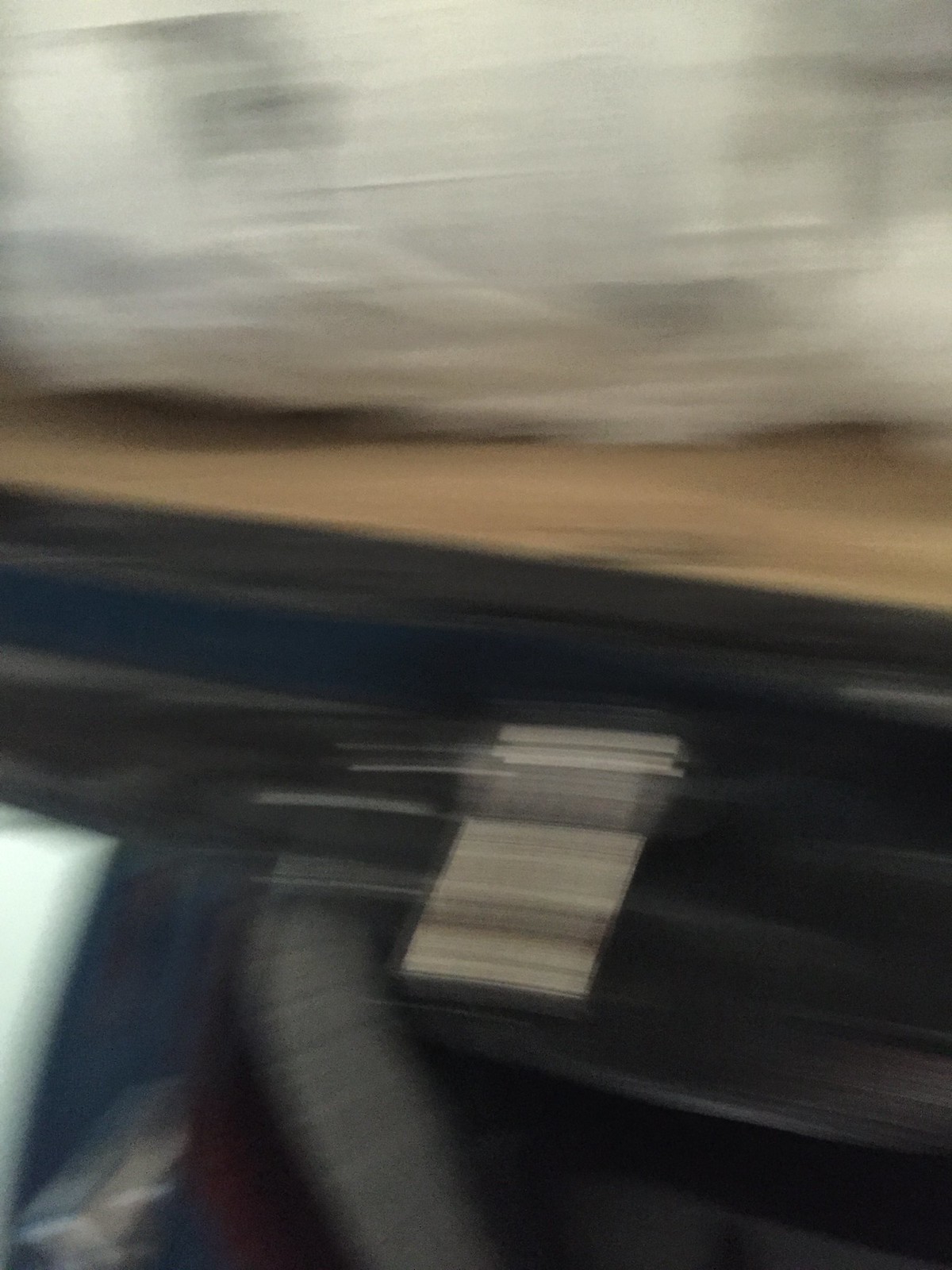The image is highly blurred, giving it a grainy and distorted quality possibly caused by erratic camera movement. Centrally featured is a conspicuously filled white bag, potentially made of canvas or plastic, resting on a surface. The bag appears to be heavily stuffed to capacity and may contain various items, lending a stretched and wrinkled appearance. It is positioned atop a beige or brown platform resembling a desk or table, possibly with fake wood texture and darker wood molding edges. Metal elements, perhaps buckles, are faintly visible, blending into the indistinguishable black surfaces that dominate parts of the image. The bottom section reveals a hint of a white object, and minor details such as a blue or black panel below the platform and an obscured limb clad in a gray and black plaid shirt, suggest a complex and somewhat cluttered environment.